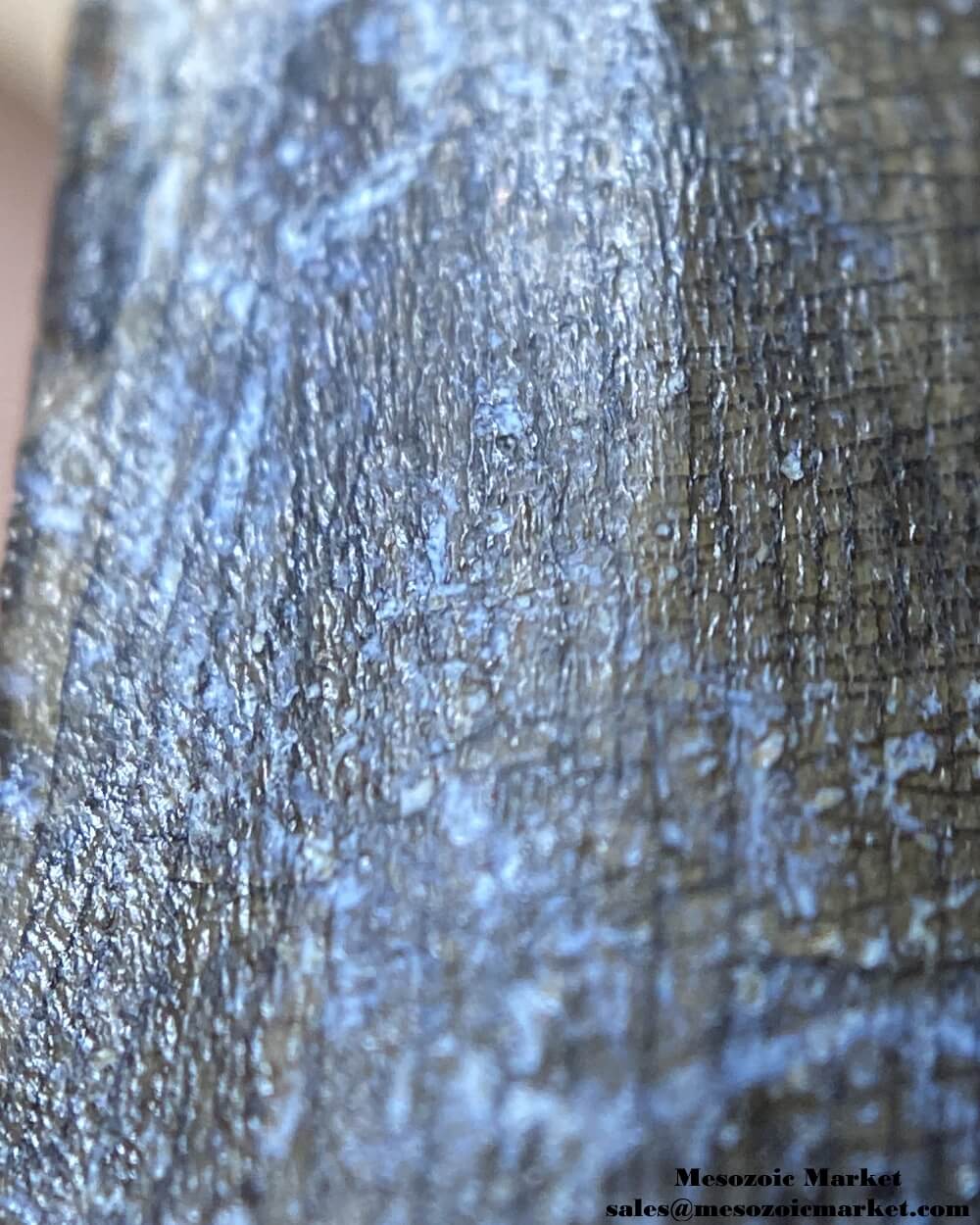This image is a detailed close-up of an unidentifiable textured surface. The surface appears shiny and gray, with hints of blue and brownish colors. It exhibits a ragged and wrinkled appearance, somewhat reminiscent of scaly skin or aluminum foil, though less smooth. The texture is bumpy, with black string-like patterns interspersed throughout. The entire frame is filled with this surface, leaving the background entirely obscured except for a tiny portion in the upper left. In the bottom right corner, small black text reads "mesozoicmarket, sales@mesozoicmarket.com". The highly magnified nature of the image makes it difficult to determine the exact material, but its appearance is almost industrial or organic, suggesting it could be something like a metallic surface or a fossilized remain.